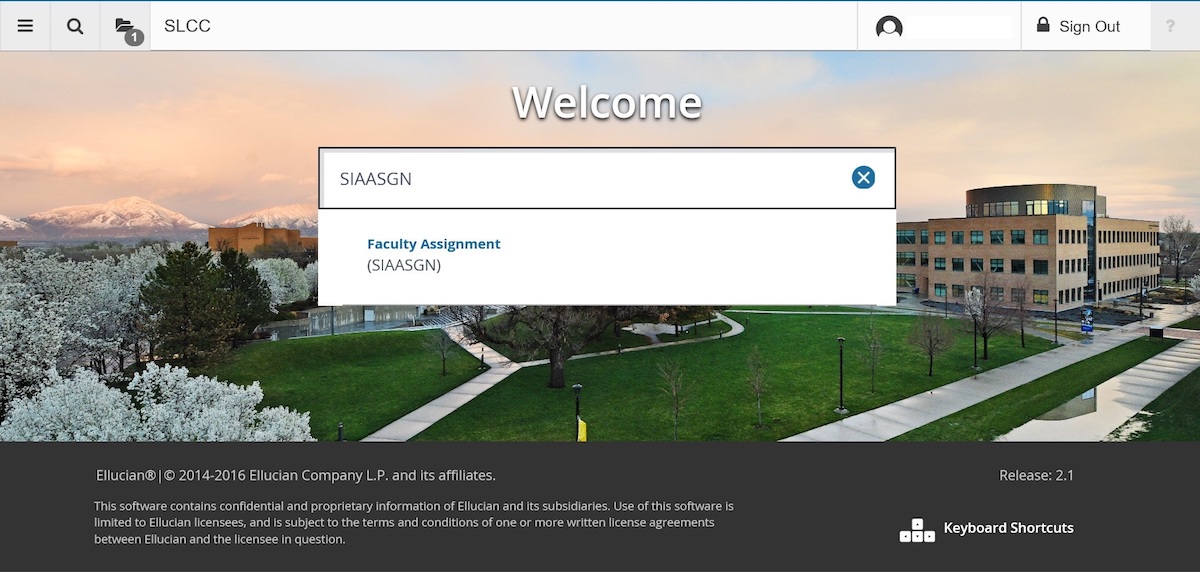A computer screen displays the Southern Louisiana Community College (SLCC) portal. The header features options for viewing one's profile and signing out, alongside a welcoming message addressed to a user named Sygen. Below this, the facility assignment is specified as Sygen as well. In the footer, the screen includes a notice indicating that the software and its content are proprietary to Ellucian Company LP and its affiliates. This software contains confidential information intended solely for use by licensed parties and is governed by specific licensing agreements between Ellucian and its licensees. The backdrop of the screen features a picturesque college campus, characterized by its historic architecture. The red-brick buildings, each standing three stories high and punctuated with numerous windows, are connected by a network of sidewalks. The campus showcases lush green expanses dotted with white flowering trees in full bloom, presenting a serene and beautiful environment.